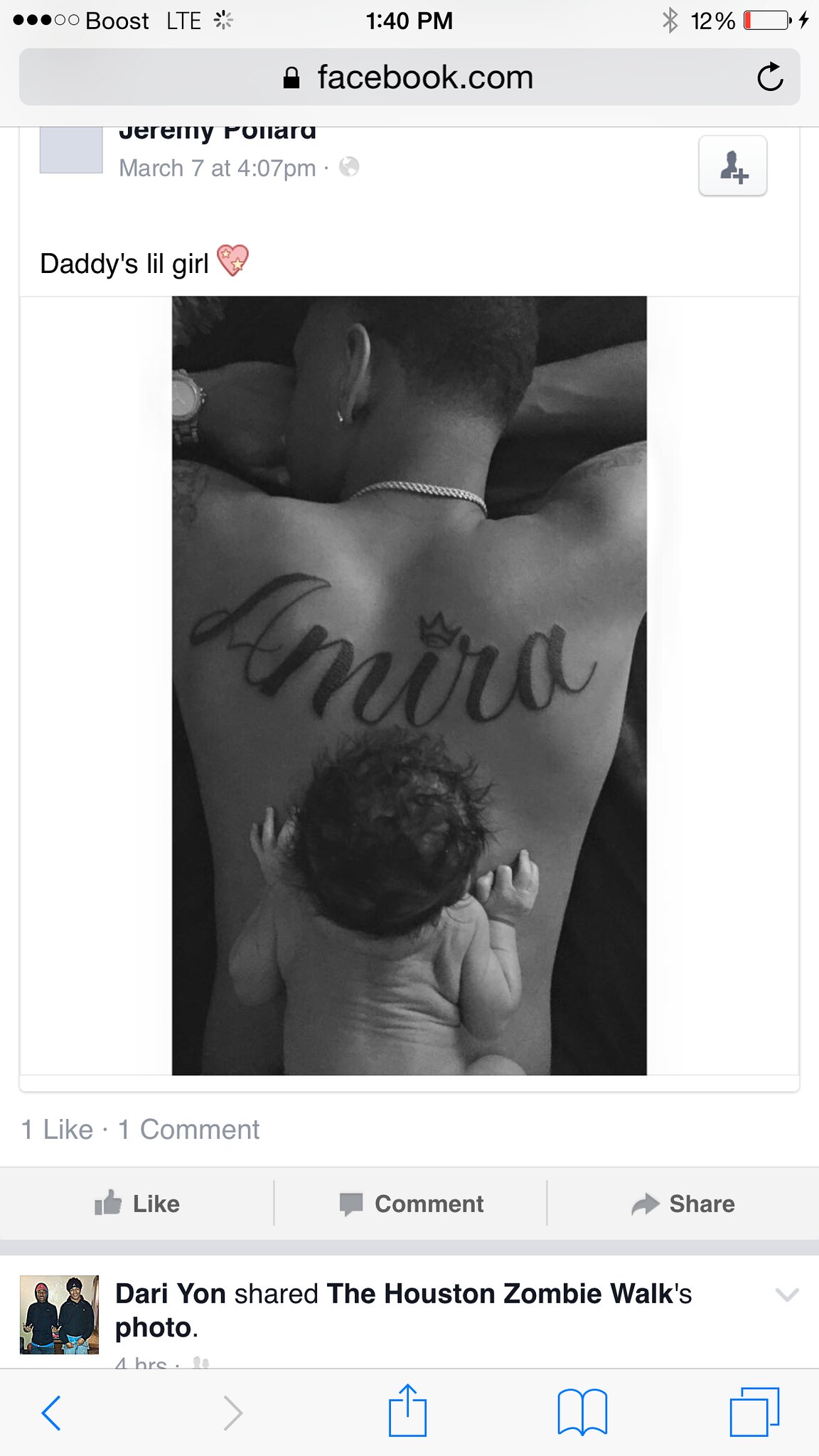The screenshot captures a Facebook post made by Jeremy Pollard on March 7th at 4:07 p.m. The phone's status bar at the top shows it is 1:40 p.m., with a Boost LTE connection, a near-depleted battery at 12% indicated by a red sliver and a lightning bolt, and a Bluetooth symbol. The browser bar underneath shows a black padlock icon beside facebook.com, with a reload arrow on the far right.

The Facebook post is titled "Daddy's Lil Girl" with a heart emoji. The image within the post depicts a man with an "Amira" tattoo on his upper back, lying on his stomach, while a baby girl is adorably sprawled across his back. The post has garnered one like and one comment, and below the image, the typical Facebook interaction options—like, comment, share—are present. Additionally, a note at the bottom indicates that Darian shared the Houston Zombie Walks photo four hours ago. The lower part of the screenshot also shows the phone's navigation buttons, including the back and home keys.